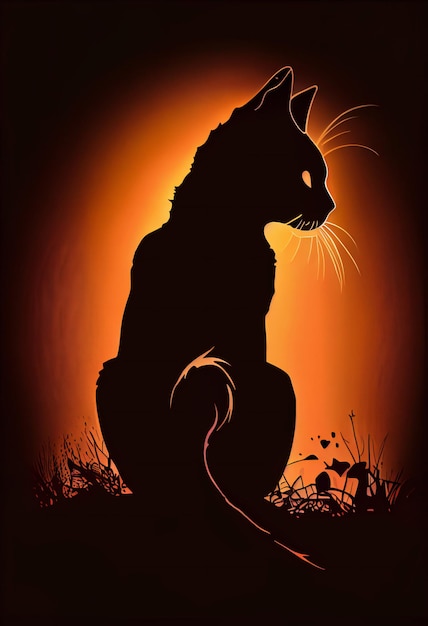The image depicts a black cat seated atop a small hill, surrounded by an assortment of weeds, tiny flowers, and grass. The cat’s distinctively curly tail, resembling a question mark, stretches alongside its body. With striking orange eyes that appear almost hollow, allowing the orange glow from the background to seep through, the cat gazes intently to the right. Highlighted by vibrant white whiskers, the cat’s slightly scruffy fur, particularly on the neck and legs, gives it a brushed appearance. The backdrop features an intense orange light, reminiscent of the glow from a fire or an oncoming train, set against a stark black background, creating a dramatic and unmistakably Halloween-inspired scene.